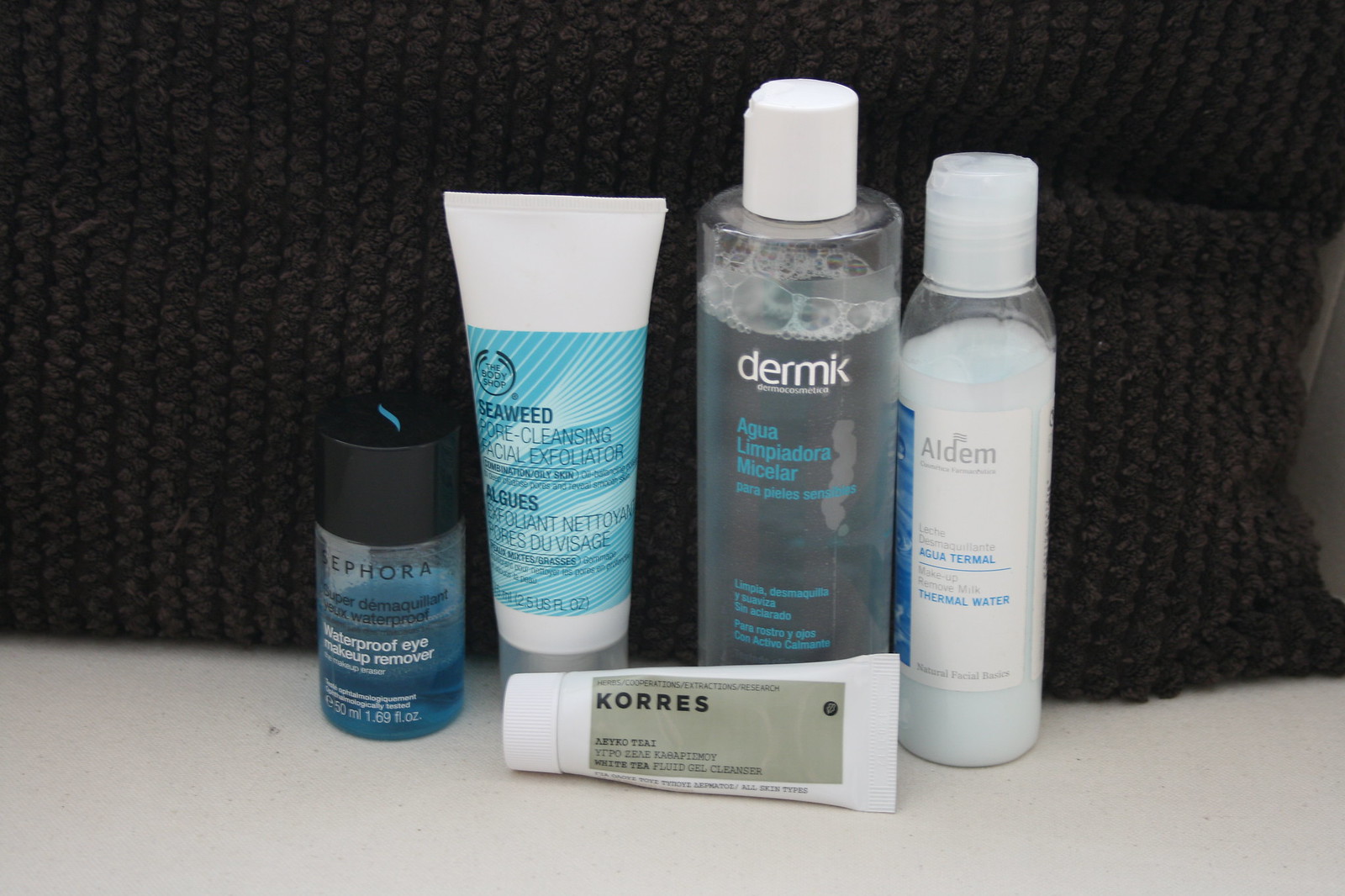The image showcases a collection of beauty products neatly arranged on a couch, positioned against a black, quilted pillow that appears hand-sewn. The main backdrop consists of the black pillow occupying the top two-thirds of the frame, with its edge curving inward about two inches from the right side before extending out of sight. The surrounding couch cushion is two-toned: gray on the sides and white at the bottom.

Starting from the left, the first item is a small plastic bottle with a black lid, accented by a blue stripe down its center. The front of the bottle displays the brand name "Sephora" in black lettering, followed by additional black and white text.

To the right of the Sephora bottle stands a tall white tube with a blue label covering about half of its surface. It is capped with a silver top. Adjacent to this is a large blue shampoo-sized bottle filled three-quarters with liquid, featuring a white lid. The bottle boasts white lettering that spells "Dermic," accompanied by blue text below it.

Next in line is a slightly shorter and slimmer clear bottle containing white liquid, with a translucent whitish cap. It features a prominent white label in the center and a partially visible blue label on its left side. 

In the foreground, lying horizontally with its cap to the left and bottom to the right, is a white squeeze bottle. It bears a gray label with the brand name "Coors" in black lettering, along with additional text beneath it.